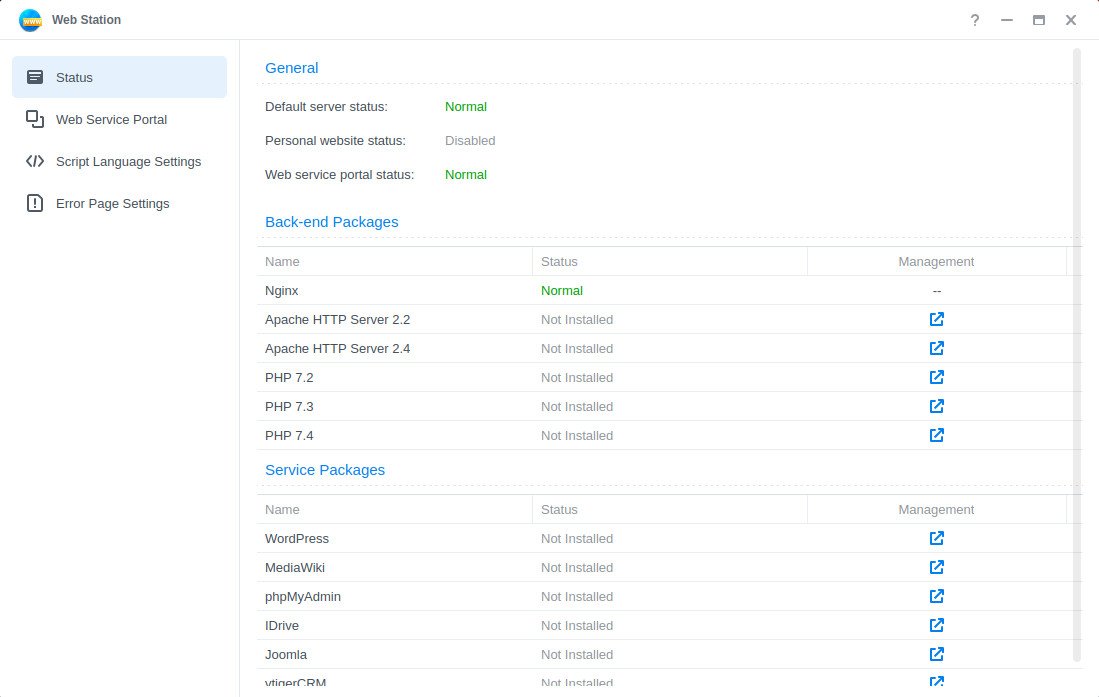The image is a screenshot of a web station interface with a clean white background. In the upper left corner, there is a round blue icon next to black text reading "Web Station." Below this header, there are several subsections:

1. **Status**:
   - **Web Service Portal**
   - **Script Language Settings**
   - **Error Page Settings**

To the right of these sections, a heading in blue text reads "General." Under this, the following statuses are listed:
- **Default Server Status**: *Normal* (in green text)
- **Personal Website Status**: *Disabled* (in black text)
- **Web Service Portal Status**: *Normal* (in green text)

Next, a blue heading reads "Backend Packages," underneath which is a table with columns "Name," "Status," and "Management." The status of various backend packages is as follows:
- **NGINX**: *Normal*
- **Apache HTTP Server 2.2**: *Not Installed*
- **Apache HTTP Server 2.4**: *Not Installed*
- **PHP 7.2**: *Not Installed*
- **PHP 7.3**: *Not Installed*
- **PHP 7.4**: *Not Installed*

Further down, another blue heading reads "Service Packages." The status of these service packages is:
- **WordPress**: *Not Installed*
- **MediaWiki**: *Not Installed*
- **phpMyAdmin**: *Not Installed*
- **iDrive**: *Not Installed*
- **Jumla**: *Not Installed*

This detailed hierarchy and status information provide a clear overview of the web station's configuration and the installation status of various packages.